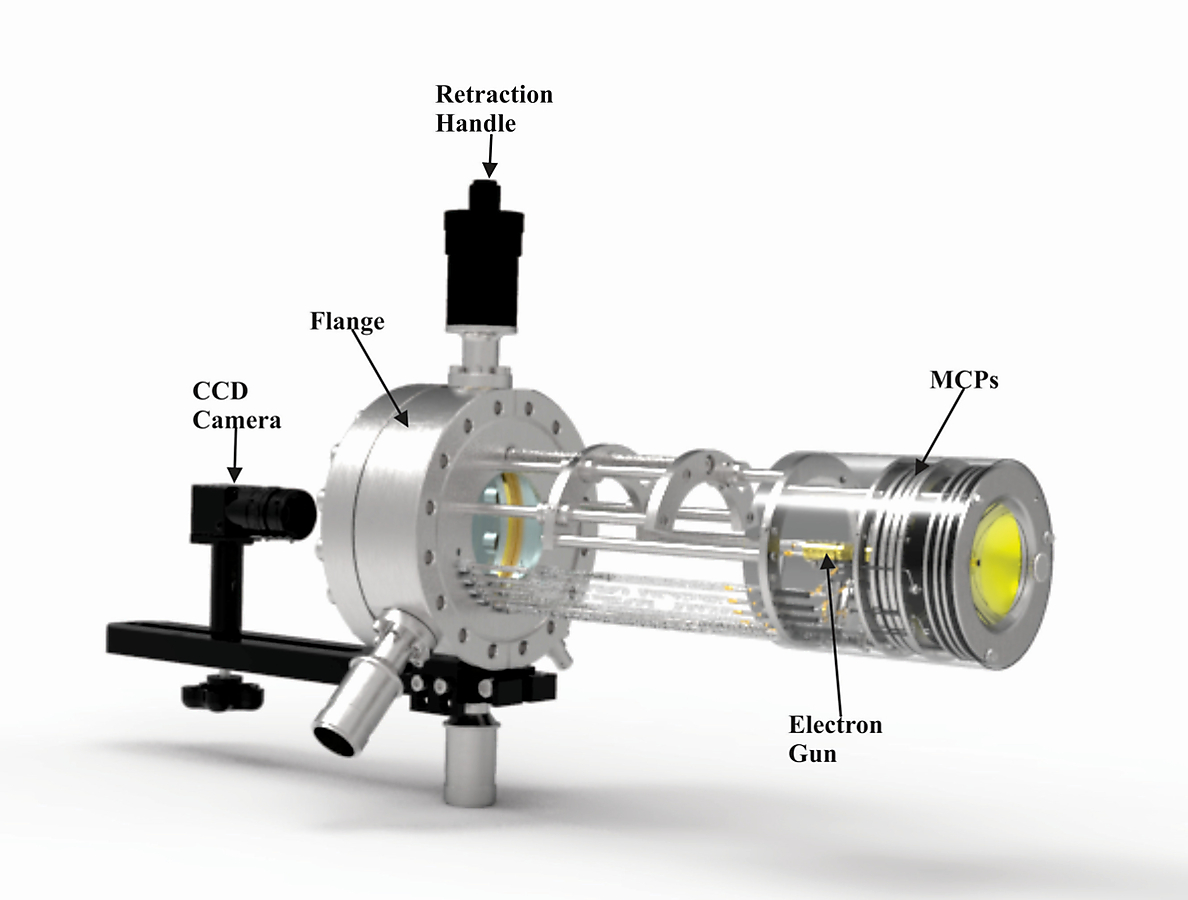This detailed photograph showcases a complex mechanical tool, depicted against a white background on a white surface with gray shadows. It is a diagram with various parts labeled. At the far left, a black line traverses the image, leading to a vertical segment with a black stem labeled "CCD camera." Adjacent to this on the right, a sizeable silver metal piece marked "flange" stands tall. Directly above the flange, a black block labeled "retraction handle" protrudes. Towards the right, stretching forward, is a cylindrical component resembling a gun barrel, which is open with visible bars and arches along its length. This transparent section features an area marked "electron gun," highlighted by a yellow lens inside. Near the top of the cylinder, a series of circular plates labeled "MCPs" (Microchannel Plates) are identifiable, adding intricate detail to the tool's structure.